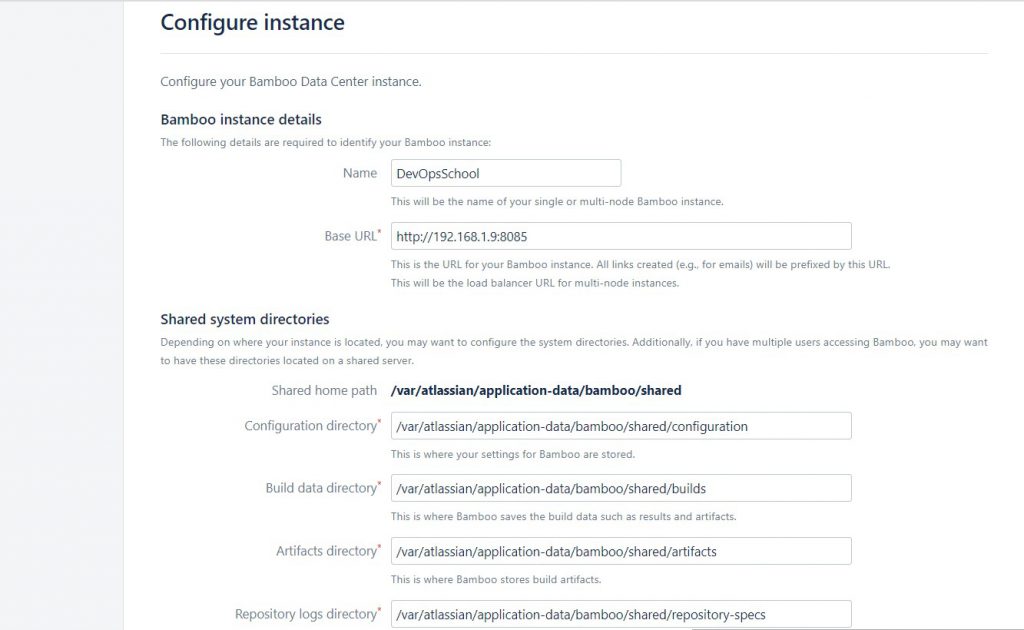**Caption:**

The screenshot features a webpage from the Bamboo software interface, commonly used in Human Resources departments. The webpage has a clean, minimalist design with a white background and a narrow, light gray border on the left side, which is empty. 

Positioned along the left edge in dark gray text is the phrase "Configure Instance," followed by a thin horizontal line. Below this, in smaller text, the instruction reads, "Configure your Bamboo Data Center Instance." Further down, a bold heading states "Bamboo Instance Details," accompanied by the clarifying text, "The following details are required to identify your Bamboo Instance."

There are two outlined input fields: the first, presently filled with "DEBOPSSCHOOL" (all uppercase and without spaces), is designated for the instance name. The second field requests a base URL, shown as an IP address.

Lower on the page, another section titled "Shared Systems Directories" appears, with additional instructions and several more outlined input fields for further configuration details.